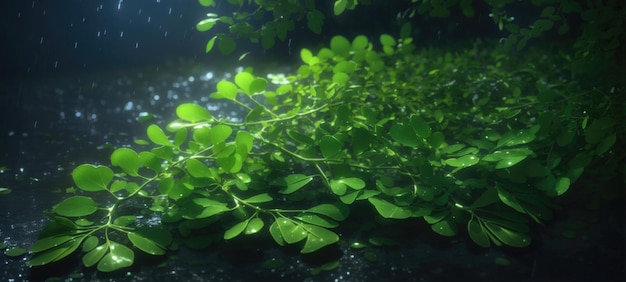This serene and calming photograph captures a close-up view of a vine with light green, abundant, smooth, round leaves, either floating underwater or resting on a glistening, rain-soaked surface at night. The background features a dark blue gradient, fading into black and dark gray, possibly hinting at a small body of water or slick soil. Speckles of light and white droplets are visible, either as rain falling gently or particles suspended in water, adding a glistening effect to the scene. The plant predominantly stretches from the right side to the center and lower right edges of the image, with another similar vine appearing in the upper section. The image is mostly dominated by the lush, healthy foliage, with any additional details in the background hazing out into darkness, emphasizing the tranquility and photorealistic quality of this night-shot, horizontal panoramic view.